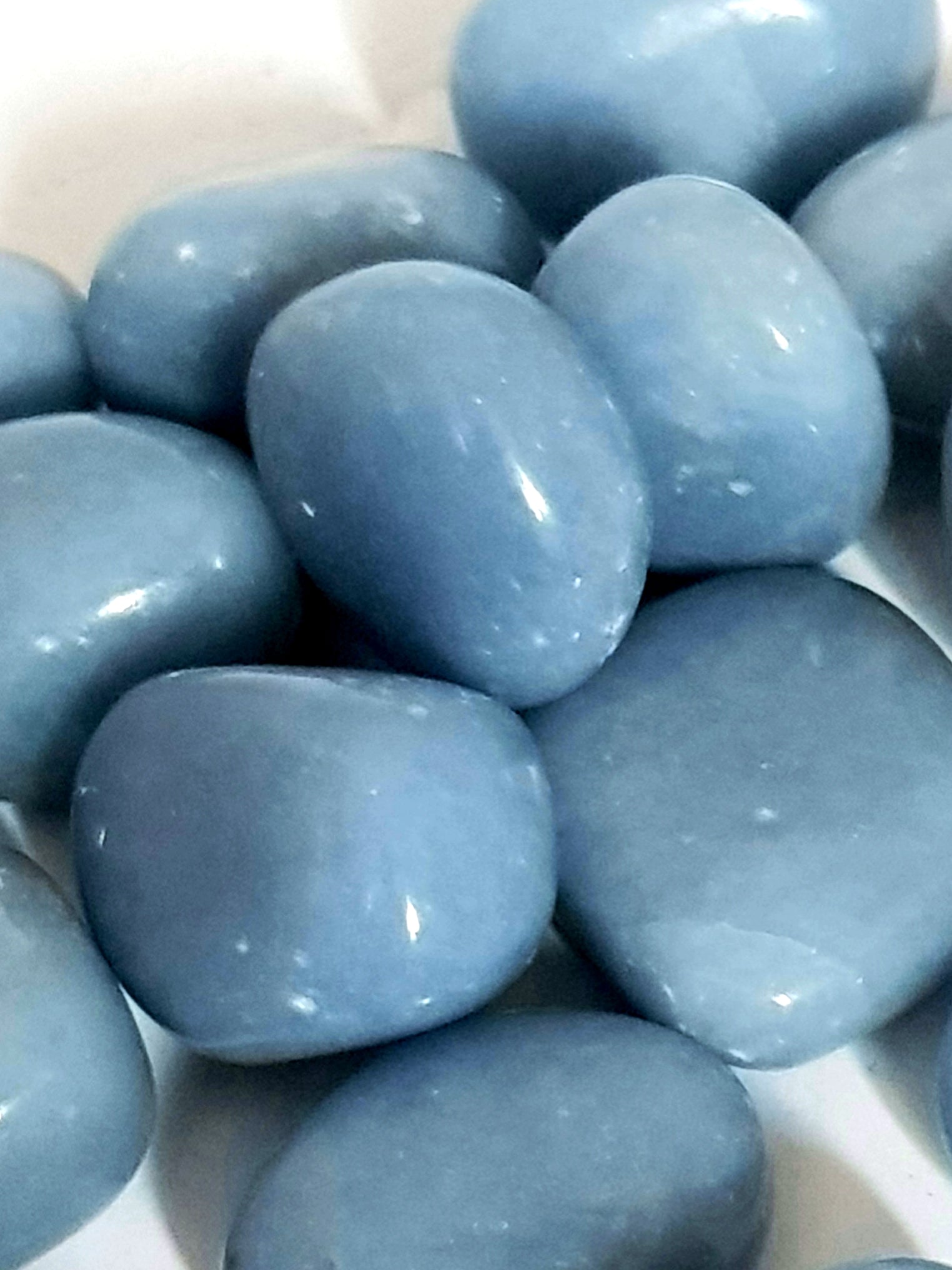This close-up image captures a dozen polished, light to medium blue tumbled stones arranged on a plain white background. The stones have an organic, river rock-like shape with smooth, rounded edges, but are not perfectly symmetrical. They are highly glossy, reflecting light and exhibiting a uniform, solid blue color without any visible markings or different hues. The stones vary slightly in size and shape, and there is a notable high polish that gives them a glossy appearance. A light source is visible, casting reflections and creating shadows between the stones. One stone at the bottom right has a small chip, providing a hint of their authenticity. The photo quality is somewhat grainy and slightly blurry, with a close-up focus that leaves only the white surface beneath the stones visible.